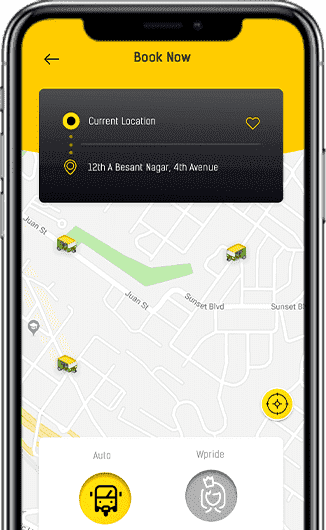The image displays a screenshot of a cell phone against a solid white background. On the left side of the phone, there are three buttons: a small one at the top, followed by two identical-sized buttons below it. The right side of the phone has a single button. At the top of the screen within a yellow box, the centered black text reads "Book Now." Below this, in a black box, the first line displays "Current Location," followed by "12th and Besant Nagar, 4th Avenue." 

The main part of the screen showcases a map primarily in shades of gray, with streets marked in white and a green area indicating a park. Notable streets include Upper Left and Wand Street on the left side, while Sunset Boulevard runs from west to east on the right. Icons resembling trucks are visible on Wand Street. The lower right corner features a compass image.

At the bottom center of the screen are two round icons: the left one is yellow, labeled "Auto," featuring an icon, and the right one depicts a princess with a crown, indicating "With Pride."